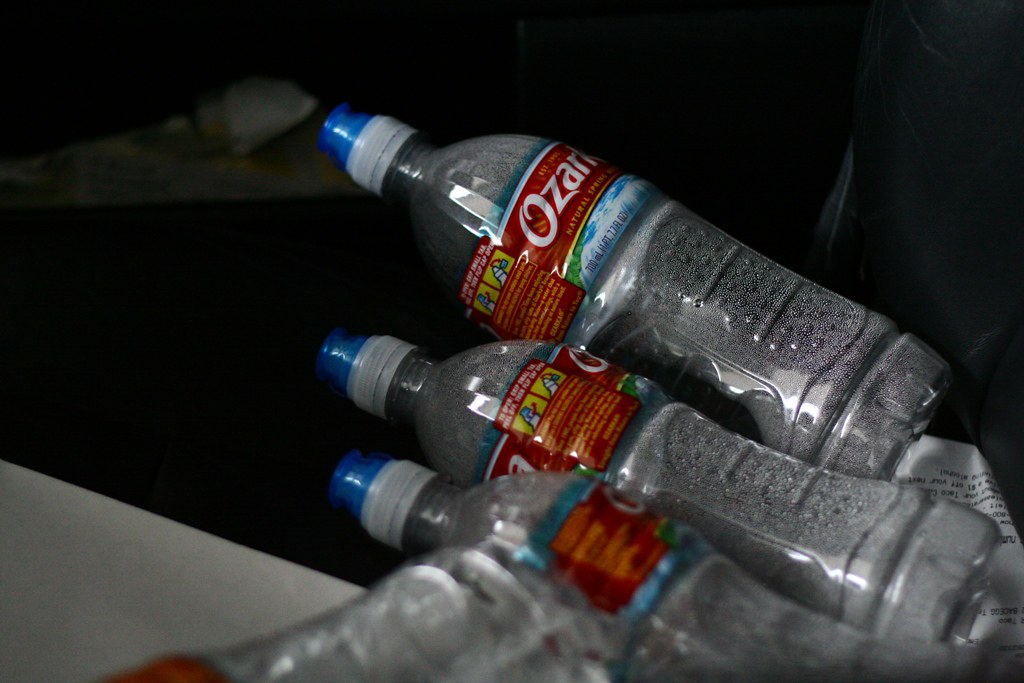The image depicts four clear, plastic water bottles with blue pop-off caps, prominently featuring red labels marked "Ozark." One of the bottles is partially cut off and blurred in the lower center of the image, while the other three are more clearly visible, although their labels are turned sideways making the full text difficult to read. All the bottles are empty, showing only condensation inside. They appear to be stacked or fallen against each other on a dark background, with a portion of what seems to be a gray surface visible in the lower left corner. The bottom right corner of the image includes a printed piece of paper positioned underneath the bottles, contributing to the sense of disarray, as if the bottles were casually discarded, likely as trash.